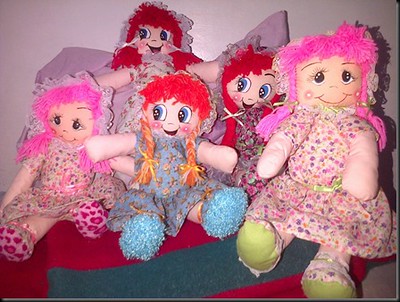In a photograph with poor lighting and a vignette effect, five Raggedy Ann-styled, soft plush dolls are seen leaning against a light lavender wall with a light purple pillow visible in the background. The dolls, adorned in vintage-style floral dresses, exhibit distinct features. Three central dolls form a triangular arrangement, each with red frizzy hair, large blue eyes, bright pink cheeks, and wide, cheeky smiles. Their hair is fashioned from yarn, with one doll in front also displaying blonde braids at the top. Each wears matching frilly bonnets and socks corresponding to their dresses. Flanking these central figures are two dolls with strikingly different appearances: they have bright pink shaggy, yarn hair, brown eyes, and similarly smiling faces. All of the dolls have rudimentary, plush arms with simple thumb-like shapes at the ends, complementing their overall charmingly cartoonish and nostalgic design.